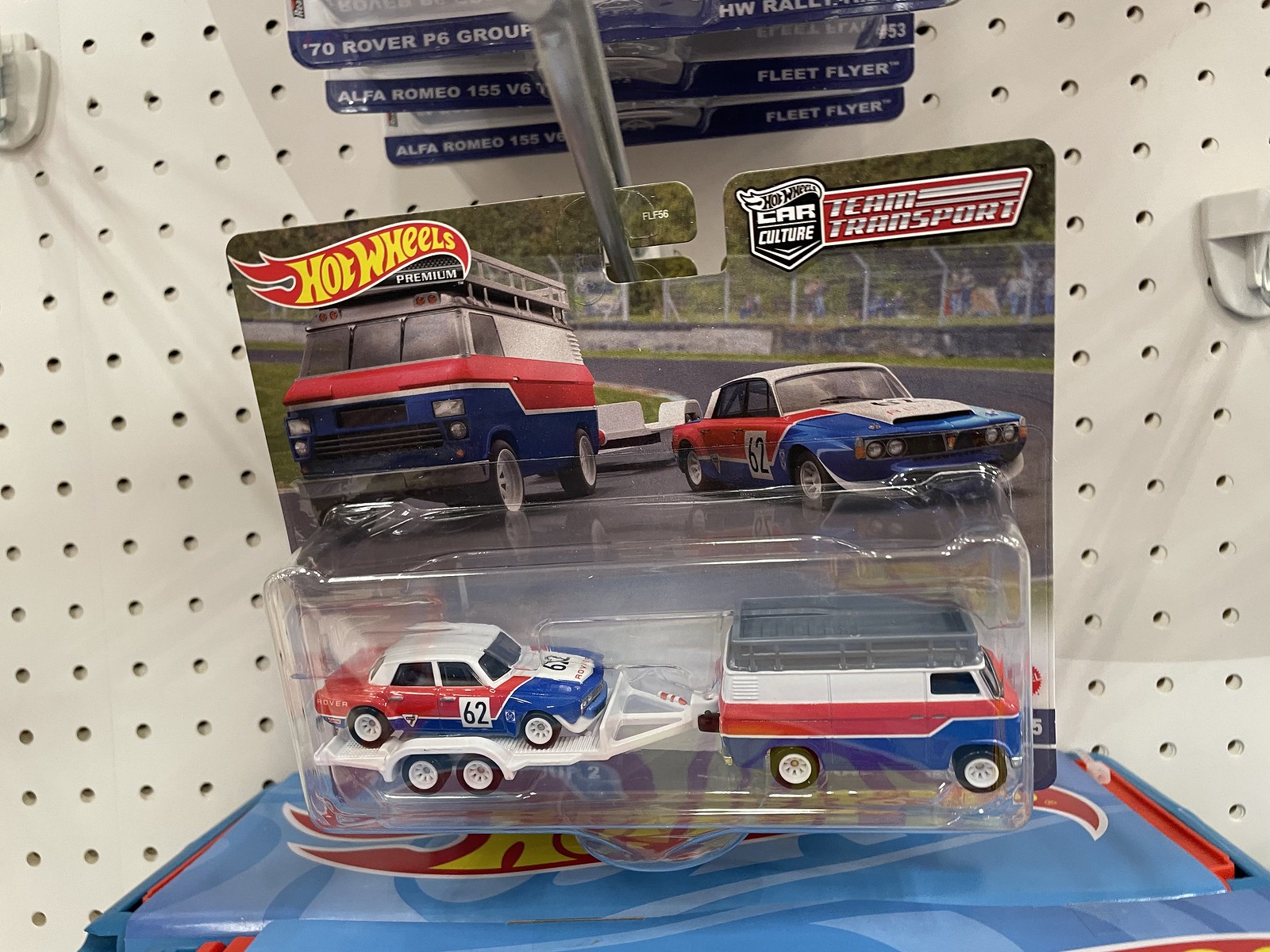The image depicts a Hot Wheels Premium Car Culture Team Transport set, displayed in a landscape-oriented color photograph against a white pegboard backdrop. The central product, packaged in shrink-wrap, showcases two meticulously replicated model vehicles. The packaging's top half features images of the actual vehicles: a red, white, and blue van on the left and a sports car on the right, both positioned on a racetrack. The sports car sports a number 62 in the middle in a racing livery. Above, a red and black logo reads "Team Transports," alongside a black shield labeled "Car Culture." Dominating the top left is the iconic Hot Wheels banner – a red flame curve with bold yellow lettering.

The lower section of the packaging, protected by bubble wrap, contains the model replicas. The front model, a van with a blue base, red middle, white top, and gray rooftop, pulls a white trailer. Atop the trailer sits the sports car, which mirrors the detailed white, red, and blue design of the actual vehicle, complete with the number 62 emblazoned on the side. The image highlights the product among a variety of other Hot Wheels models hanging from the pegboard, emphasizing its intricate, realistic details and vibrant color scheme.